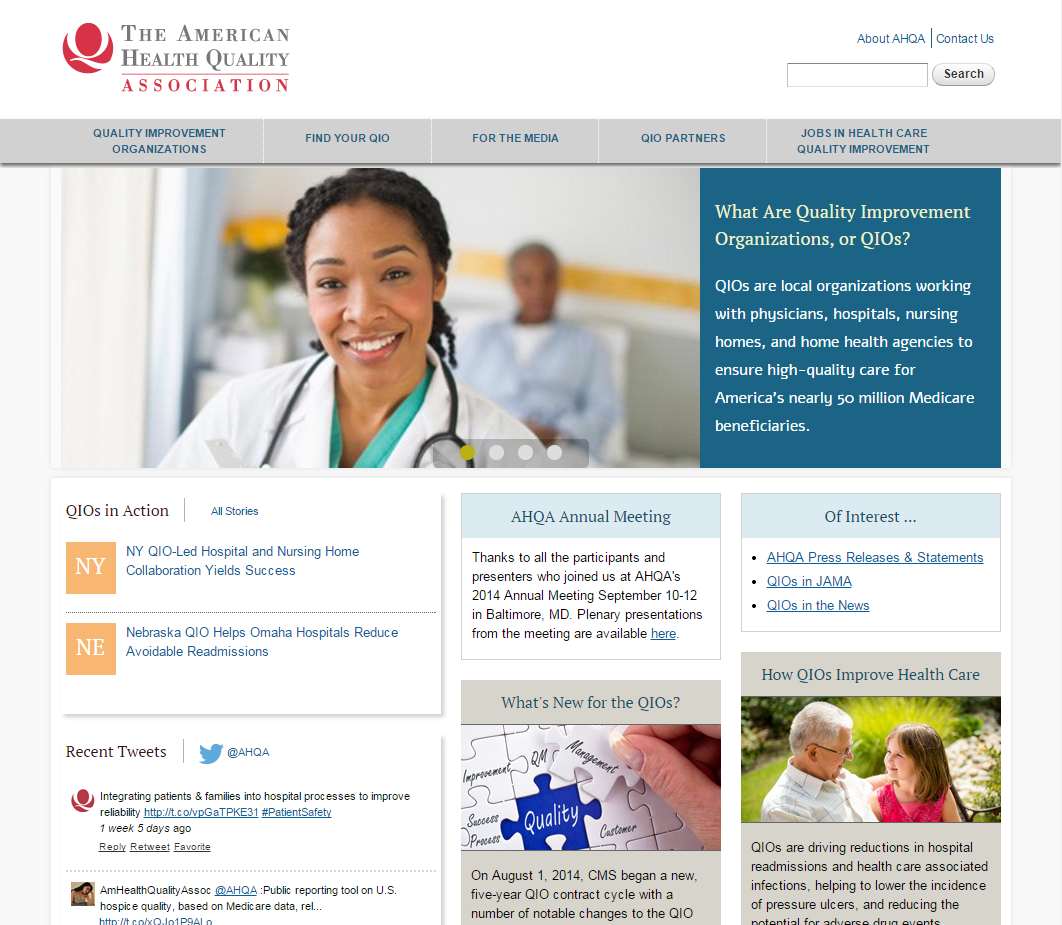Screenshot of the American Health Quality Association (AHQA) Website

The screenshot captures the homepage of the American Health Quality Association (AHQA) website. Dominantly featured at the top is the AHQA logo in red with a red line above it, while the rest of the text appears in gray serif font. To the left of the logo is a decorative element: a white "Q" enclosed in a red circle, with the top and right edges of the "Q" extending beyond the circle's boundary.

In the upper right section of the page, there are navigational links labeled "About AHQA" and "Contact Us," along with a capsule-shaped search button and field. Below the header, a gray menu bar lists several categories: "Quality Improvement Organizations," "Find your QIO," "For the Media," "QIO Partners," and "Jobs in Health Care Quality Improvement."

Central to the page is an image showcasing an African-American female doctor with a stethoscope and a white lab coat, partly covering blue and green scrubs. She has braided hair pulled back and is seen smiling warmly at a blurry patient lying on a bed in the background.

Beneath the image, four photo option circles are displayed – one in yellow on the far left and the other three in white. Adjacent to these circles on the right side is a blue square with textual content explaining "What are Quality Improvement Organizations (QIOs)?" It states: "QIOs are local organizations working with physicians, hospitals, nursing homes, and home health agencies to ensure high-quality care for America's nearly 50 million medical beneficiaries."

The lower left of the page includes options for different states, such as New York and Nebraska, and showcases recent tweets. Additionally, four panels on the right-hand side provide information about the AHQA annual meeting and feature other relevant updates.

A map indicating "What's New," along with various links of interest, is also visible. An image of an elderly man, possibly a grandfather, with a young boy beside him, suggests how QIOs are improving health outcomes, particularly by driving the reduction of hospital admissions.